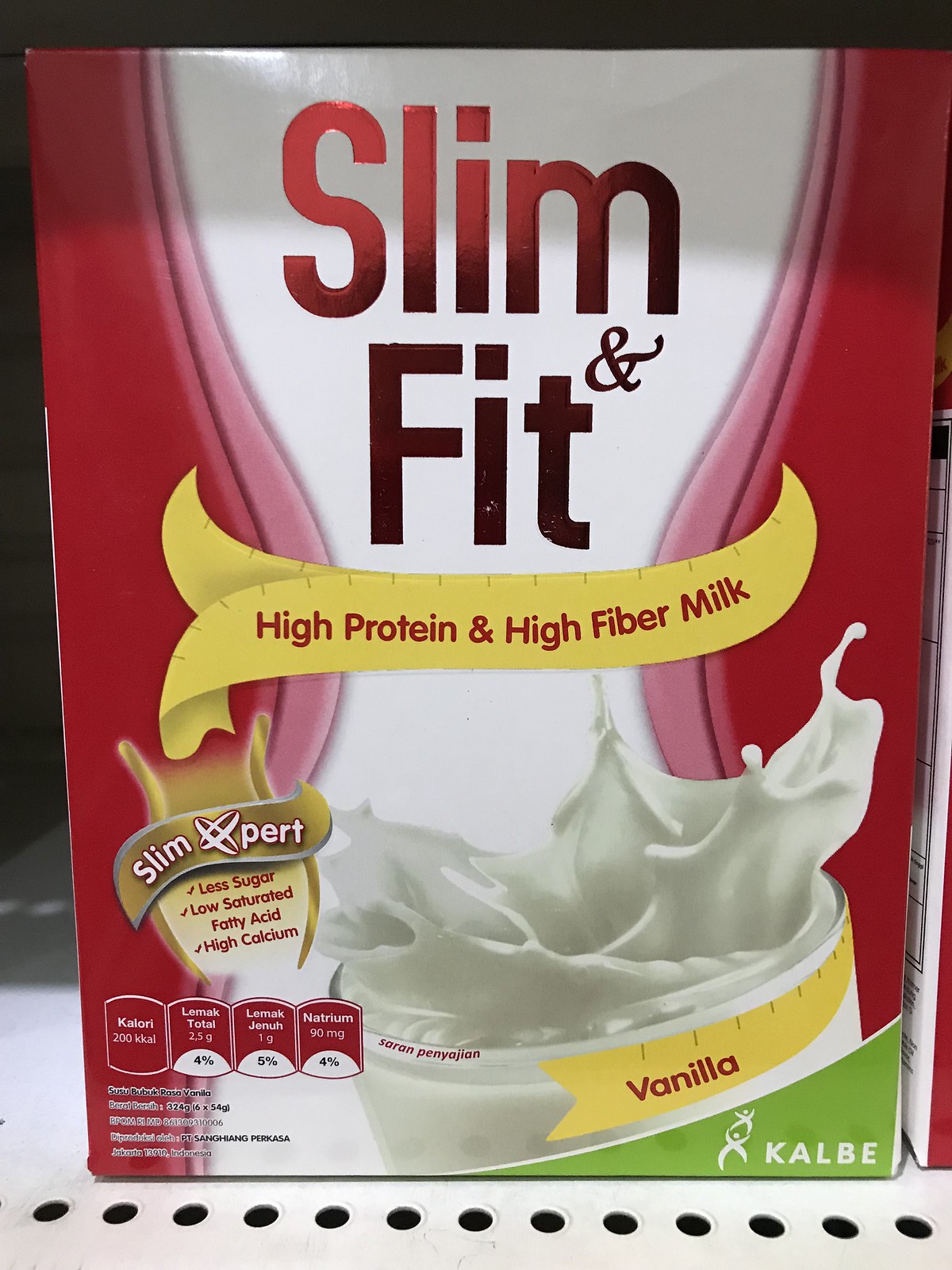This portrait-style photograph captures the packaging of a protein shake mix on a store shelf, as indicated by the characteristic white shelving. A partially visible, similar package on the right edge hints that this product is displayed alongside other identical or similar items. The packaging is a box with the product name "Slim and Fit" prominently displayed in a metallic red sans-serif font. Beneath the name, a yellow banner with a ribbon-like design bears the product description in red text, highlighting its benefits as a "high protein and high fiber milk." Additionally, the bottom right corner features the flavor "vanilla" in a green curved cutout, accompanied by a logo for a different service and the name "K.A.L.B.E."